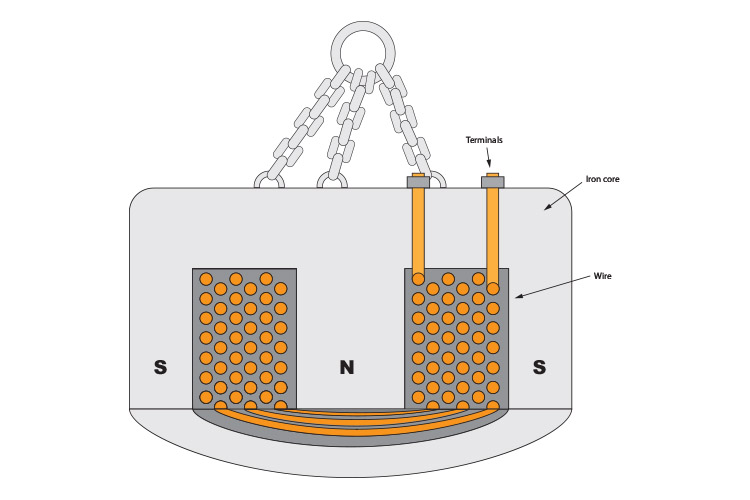The diagram features a white background with a gray circle at the top, from which three gray chains hang. The left chain extends diagonally outwards, the center one also leans slightly to the left, and the right chain hangs straight down. These chains are connected to a light gray rectangular object with an arched bottom, which is also outlined in gray. This rectangle is divided into three labeled sections: 'Terminals,' 'Iron Core,' and 'Wire.'

The 'Terminals' section is located at the top and features a small gray square capped by a yellow square. The 'Iron Core' takes up the central area of the gray rectangle, while the 'Wire' section includes two dark gray vertical rectangles filled with dark yellow dots, and are marked with letters 'S' at the left, 'N' in the middle, and another 'S' on the right. These letters are positioned between the yellow dots. Black arrows point downward, directing attention to these sections. Additionally, there are slanted gray and yellow lines repeated at the bottom of the image. This diagram resembles a battery held up by three chains, illustrating the components and their functions.